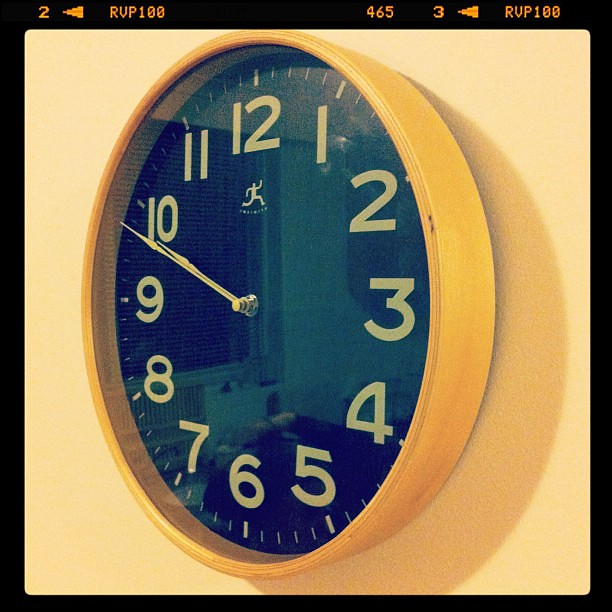The image features a vintage-style clock with a yellow-orange body, facing slightly to the left. The clock has a striking black face adorned with white numerals ranging from 1 to 12. A unique detail on the clock face is a small white graphic of a running person, likely representing a logo. Beneath this logo is some indistinct, small text.

The clock’s two silver hands are positioned just below the 10 o'clock mark. Covering the clock face is a glass panel, casting a reflection that includes a window and a section of what appears to be a kitchen area, with yellowish walls in the background.

Overlaying the image is a user interface displaying various elements. In the top left corner, there's a number "2" and a left arrow. Beside these, "RVP 100" and "465" are noted, followed by another digit "3" and a yellow arrow pointing to the left. This UI annotation repeats the text "RVP 100."